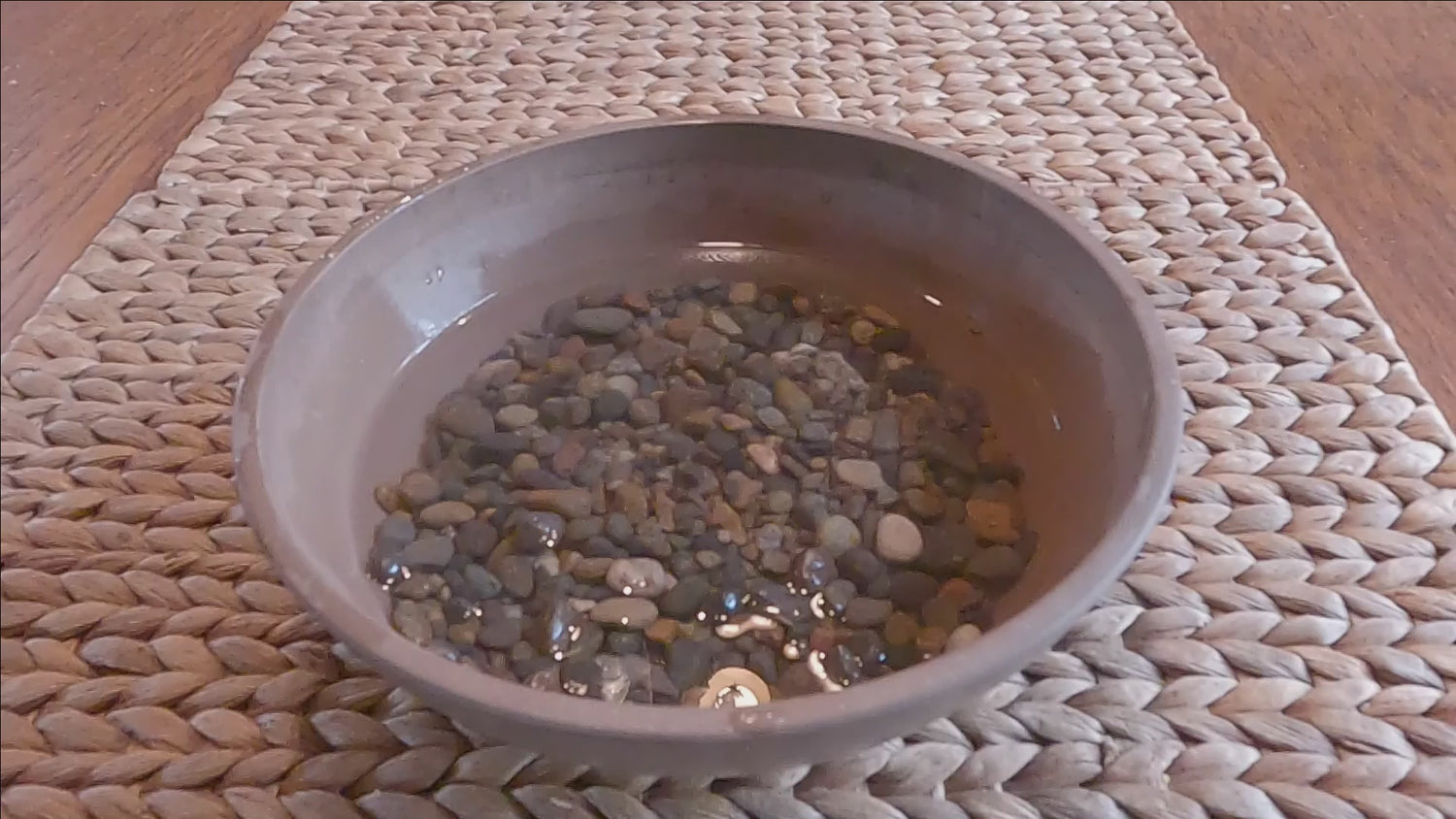The photograph captures a large, shallow gray bowl, possibly made of plastic, partially filled about a quarter way with water. Within the water, a diverse collection of small, smooth pebbles and decorative stones rest, showcasing an array of colors including white, gray, black, brown, and shale. The water level is low, just enough to create a subtle reflection of a nearby lamp on the water's surface. The bowl itself is placed on a long, rectangular off-white woven placemat, which lies on a wooden floor, adding an indoor setting to this aesthetically arranged display. The stones, reminiscent of those used in decorative plant vases, collectively amount to well over a hundred, creating a textured and colorful composition beneath the water.